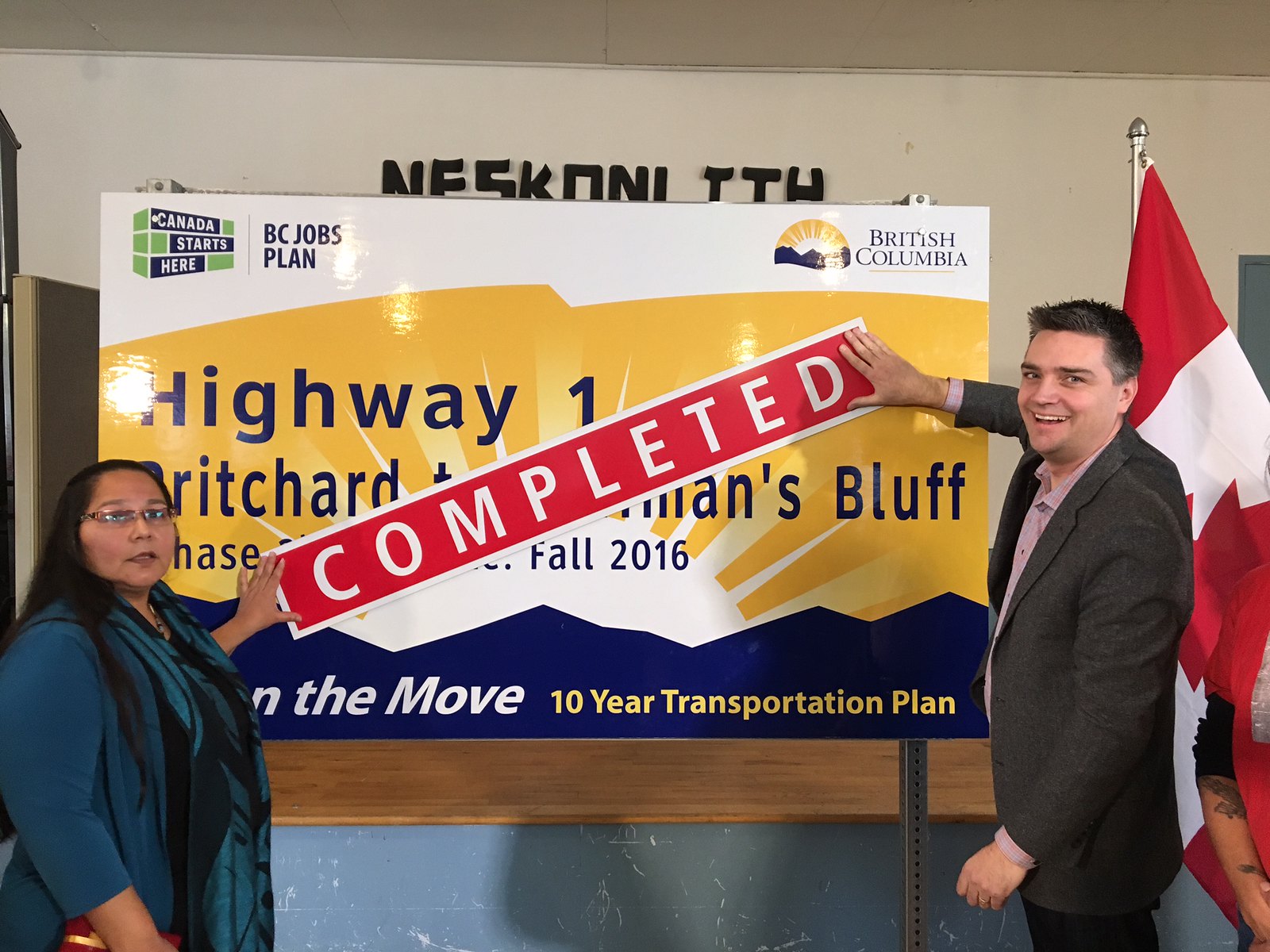In the image, two people are standing in front of a large sign inside an office building with white walls and cut-out black lettering partially obscured by the sign. The foreground features a prominent sign with multiple sections. In the upper left, it states "Canada Starts Here" and, to the right, "BC Jobs Plan" in blue font. The upper right corner reads "British Columbia" alongside its icon. The sign has a yellow section with bold blue letters spelling "Highway 1" and partially visible text that says "Pritchard," "MANS," and "BLUFF CHASE." Additional details mention "Fall 2016," "ON THE MOVE," and "10 Year Transportation Plan."

In front of this sign, a woman with dark brown hair in a green, flowy formal outfit stands on the left, and a man in a gray suit jacket smiles at the camera on the right. Both are holding a red, diagonal sign with white letters spelling "COMPLETED," covering parts of the background text. To the right of the man, a Canadian flag on a silver pole is partly visible, contributing to the celebratory atmosphere of a completed project, likely part of the 10-year transportation plan.